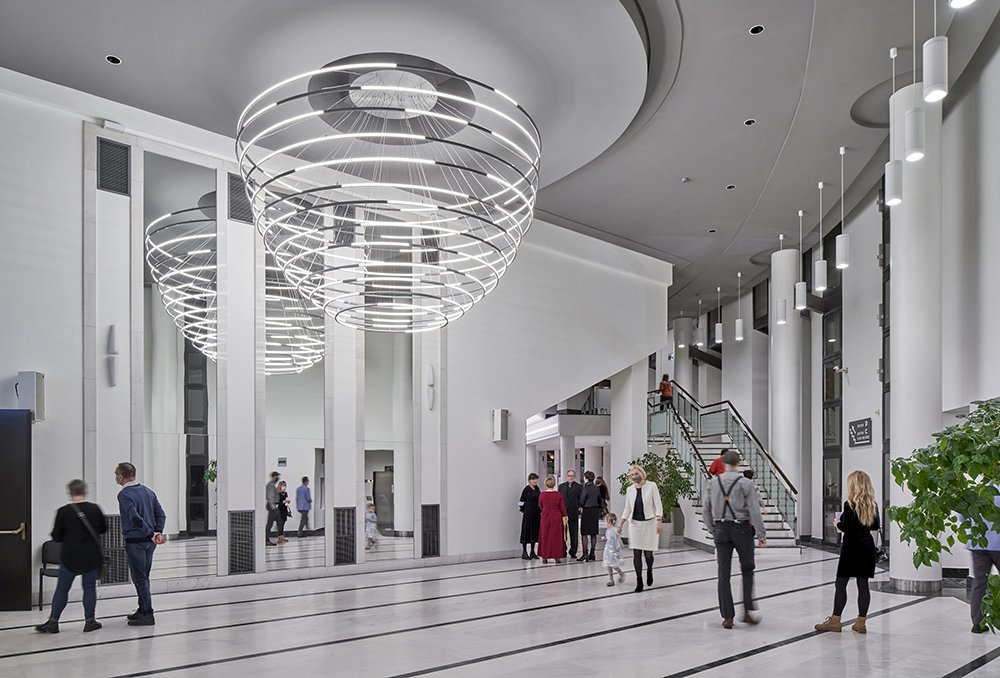The image depicts the expansive lobby of a building that could be an apartment complex, office building, or a fancy hotel, characterized by its modern and New Age design elements. The room is incredibly spacious with very high ceilings, accentuated by white marble floors with black stripes and light gray walls, giving it a clean, minimalist look. Dominating the ceiling are two distinctive chandeliers, each resembling the rings of Saturn in descending order and enhanced by spiral light designs, one of which is reflected in a mirror adding dynamic visual interest. The right-hand side of the room features a grand staircase and is lined with numerous spotlights. Additionally, there are several planters with tall green trees adding a touch of color. Scattered throughout the room are groups of people including a man in overalls, a man dressed in blue, a woman in a pantsuit holding a child’s hand, and a young blonde woman in black gazing up the staircase. The overall ambiance is one of elegance and modern sophistication.